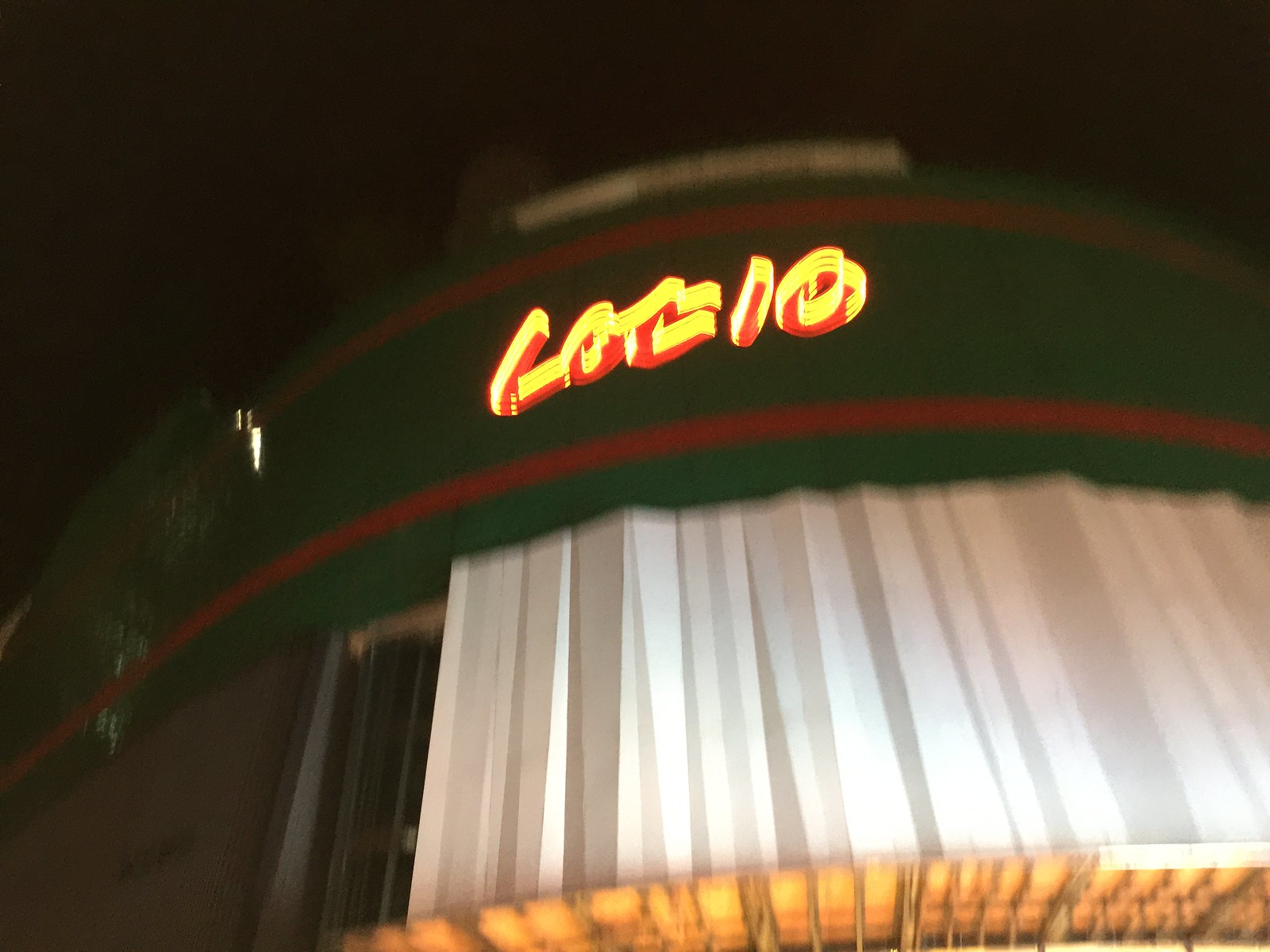This photograph features a nighttime scene that is somewhat out of focus, creating a slightly mysterious and indistinct visual. The primary subject appears to be a building with an arched, curved facade. Prominently displayed at the center of the building is a sign, which partially reads "L-O-...I-O," though the remaining letters are unclear. Beneath this sign, elements resembling a harlequin's collar—folded white shapes arranged in a curved pattern—add to the enigmatic quality of the scene. The overall lack of sharpness and the dark atmosphere contribute to an intriguing, almost surreal visual experience.